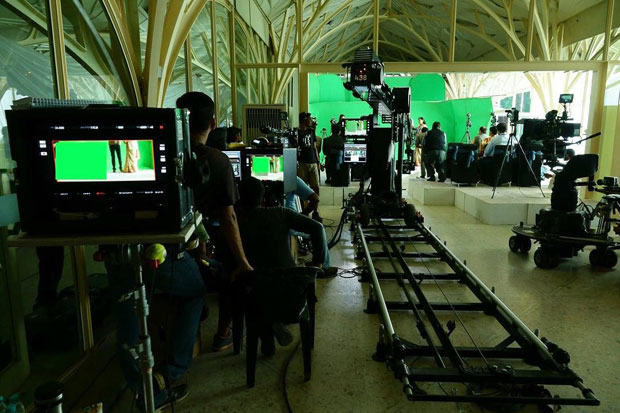The image depicts the interior of a bustling studio. In the foreground, a black camera on a metal track occupies the right side, capturing the scene toward the stage. The stage itself, positioned in the background, is bathed in sunlight from the left-hand side, contrasting with its white surface. A man in a black t-shirt with dark hair stands in front of the camera, intently observing the stage. On the stage, a group of people is visible against a backdrop of green walls; one man faces away while another faces forward. Various black cameras are strategically placed around the studio, some mounted on tripods, others on metal tracks, and a few on wheels. The roof above is a wooden lattice, covered with a white layer, allowing natural light to fill the space. The setup hints at a lively production environment, with equipment scattered between the foreground and the stage, emphasizing the dynamic and industrious atmosphere of the studio.